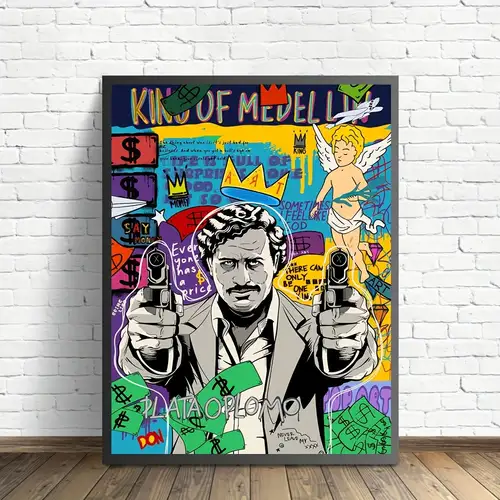This image depicts a graffiti-style poster leaning against a white brick wall on a light wooden floor with a wood baseboard. The rectangular poster has a dark grey border and features an elaborate black and white drawing of Pablo Escobar in the center. Escobar is illustrated with curly black hair, a mustache, a suit coat, and a white shirt, holding two pistols pointed outward. Green dollar bills with black dollar signs are scattered around him, particularly in the lower left and right corners, and small boxes with dollar signs ascend from the gun in his right hand. Above him, the text "King of Medellin" is prominently displayed, with a green dollar sign integrated into the word "King" and a red crown over the "ED" in "Medellin." The red and yellow crowns also appear above and to the left of Escobar's head, where faint purple graffiti text is visible. Additionally, a childlike angel with yellow hair, white wings, and a diaper is illustrated on the top right of the poster. The image is vibrant with graffiti-style elements and various graffiti texts scattered throughout, contributing to its dynamic portrayal of Escobar.